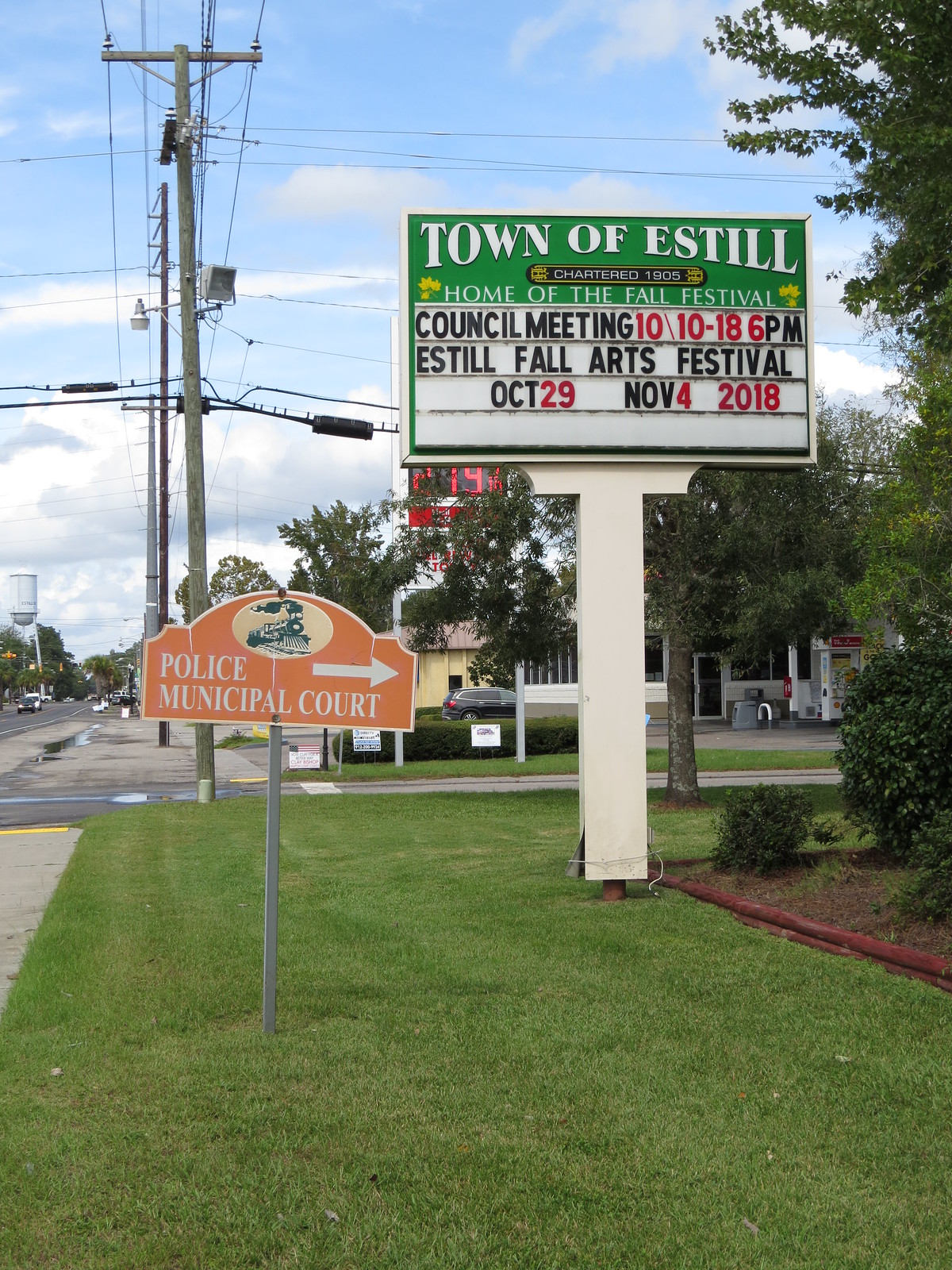The image showcases a vibrant town scene centered around a prominent "Town of Estill" sign, indicating the town's establishment in 1905 and promoting local events such as the Fall Festival and council meetings. The sign is predominantly white with green and black text, accented by red numbers. Below and to the left of this main sign is a smaller, light orange sign directing to the Police Municipal Court, adorned with an image of a train. 

The foreground features a well-maintained lawn of light green grass, surrounded by lush greenery including trees and bushes. The bottom half of the background on the right side includes a gas station with a black car parked nearby. A long street extends from the middle to the left side of the image, hosting several cars and leading towards a distant water tower painted light blue. The setting is bathed in daylight with a partly cloudy sky overhead, blending soft whites and blues, creating a serene and picturesque small-town atmosphere.